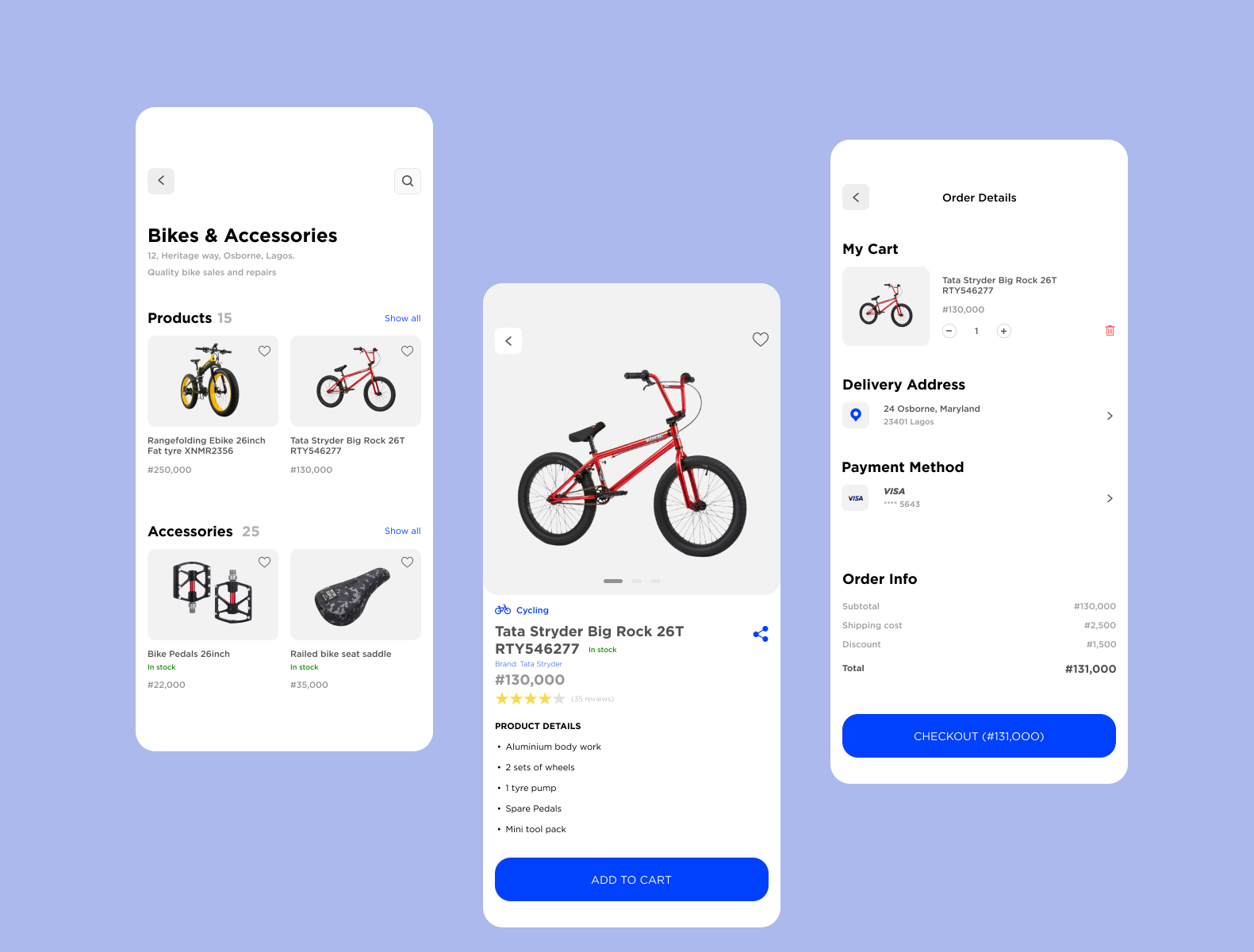The image features a large blue box containing three distinct phone screen displays, each illustrating different stages of a shopping app. 

The first screen showcases a section titled "Bikes and Accessories," listing a total of 15 products. Within this section, a grid of four images is visible. The first two images display bicycles: one bike has a striking yellow rim against an all-black frame, while the other boasts a vibrant red frame paired with black wheels. Additionally, there are two accessory tiles in this section, highlighting bike pedals and a bike seat. Below these images, clickable "See All" hyperlinks invite users to explore more bikes and accessories, which total 25 items in the accessories category.

The second screen centers on a specific bike, identified as a Tata Schrader Big Rock 26T. This bike, previously seen in the first screen's product list, is depicted with its red frame and black tires. Beside the image, the bike's serial number and a price tag of $130,000 (likely in a non-American currency) are displayed.

The third screen shows the user's shopping cart, containing the Tata Schrader Big Rock 26T. Details include order specifics such as the delivery address, payment method, subtotal, any applicable discounts, and the final total. A prominent blue button labeled "Checkout" is available for proceeding with the purchase.